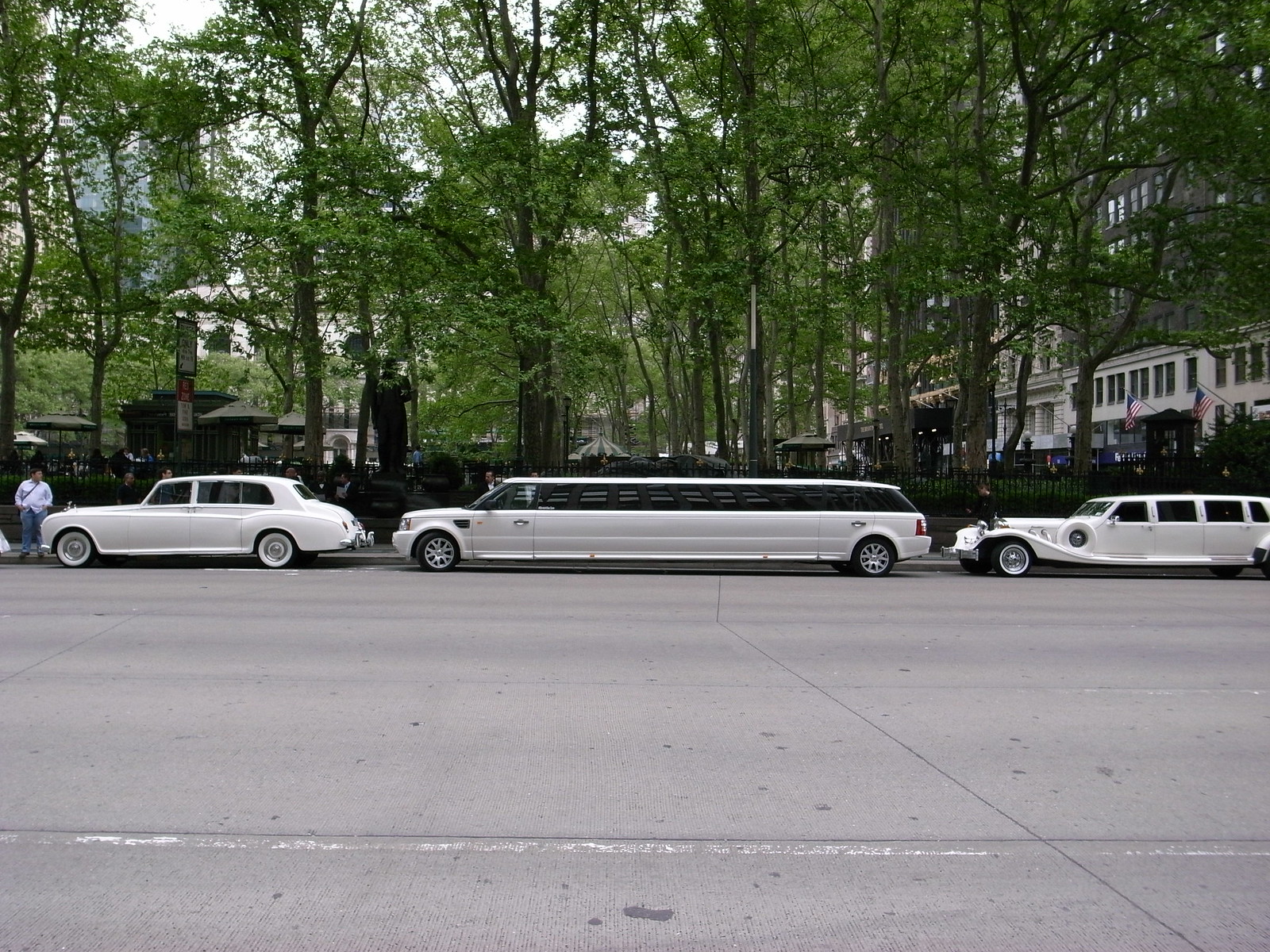The photograph is a split image with the bottom half in black and white and the top half in color. It features a bustling city square, possibly in Manhattan or London, with three white luxury cars—likely a Bugatti, a Rolls Royce, and a stretch limousine—parked in a line from right to left on a gray pavement street. The limousine is centrally located, flanked by the other two vehicles. The cars have dark, almost black, window areas. Behind them is a wrought iron fence typically found in upscale urban areas, enclosing a small park with several trees. To the right of the image, adjacent to the third car, is a white building adorned with two American flags. The park’s foliage is lush, providing ample shade, and part of the sky visible at the top is a blue-white hue. On the left side, a man in a white shirt, jeans, and a shoulder bag is standing. The street extends alongside the park, bordered by additional buildings and more leafy trees, creating a picturesque urban scene.